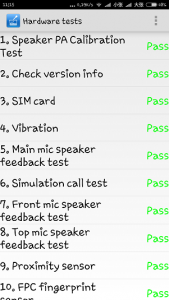The image is a vertically-oriented rectangle, resembling a screenshot captured from a smartphone. At the top, a black bar displays standard phone icons for Wi-Fi, signal strength, battery status, and cell service, but the text appears in an unusual, almost handwritten font. Directly below this black bar, another section, labeled "Hardware Tests," appears, featuring a blue box on the left side and a vertical three-dot menu icon on the right.

Beneath this, a list of ten hardware tests is presented, each item separated by a thin gray line. All tests are marked with a green "PASS" indicator on the right-hand side. The tests are as follows:
1. Speaker PA Calibration Test
2. Check Version Info
3. SIM Card
4. Vibration
5. Main Mic Speaker Feedback Test
6. Simulation Call Test
7. Front Mic Speaker Feedback Test
8. Top Mic Speaker Feedback Test
9. Proximity Sensor
10. FPC Fingerprint